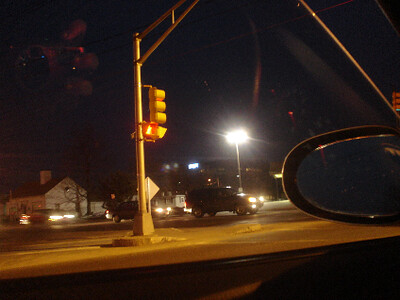A nighttime photograph captured from the driver's side window of a car stopped at a traffic light. The image includes part of the car's rearview mirror, window frame, and door frame. Ahead, a crosswalk signal mounted on a silver pole glows red, nestled within a curve on the street. A yellow traffic light signals red, overseeing the cross traffic. The scene features several vehicles: a red car, a gray car, and a black car, all with their headlights illuminated. The sky is a deep black, with a single bright street lamp casting light over the intersection.